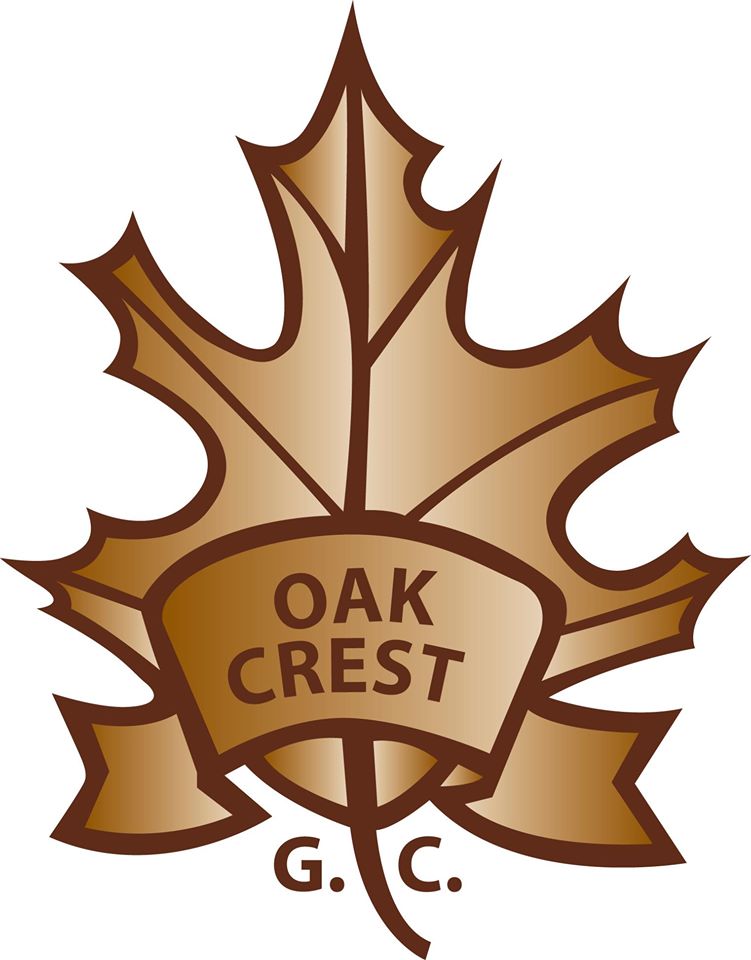The image depicts a detailed logo or crest set against a white background, creating the illusion that it is floating in a white void. The central element is a large, stylized leaf with seven ridged spikes—three on each side and one central spike. Each spike features lines running down its length. The leaf has a gradient brown color scheme, starting as a lighter brown in the center and darkening towards the edges, where it is outlined in dark brown. In the center of the leaf, there is a rounded banner with dark brown text reading "Oak Crest." Below the leaf, the stem extends downward, flanked by the letters "G" and "C" at its base, also in dark brown. The meticulous shading and structure give the logo a polished, almost translucent appearance.